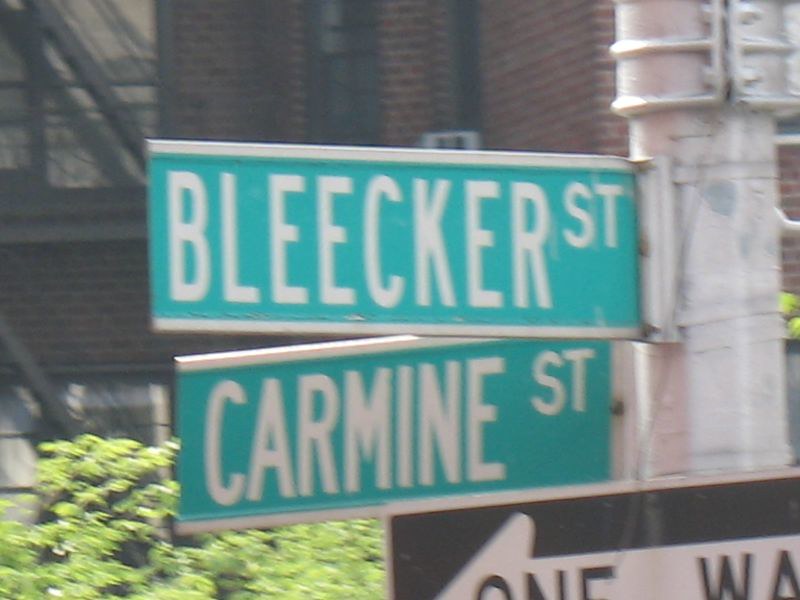In the foreground on the bottom left, vibrant green leaves add a touch of nature to the scene. The setting features an encompassing background of brick walls, marked with windows in the top left corner, through which hints of staircases are visible. Dominating the right side of the image is a central pole. Positioned on the bottom right is a distinctive one-way sign: a black rectangle with a white arrow pointing left and the words "One Way" in black text. Above this sign, a green street sign displays "Becker Street" in white text, while a second line of white text shows "Carmine Street," offering clear navigational cues.